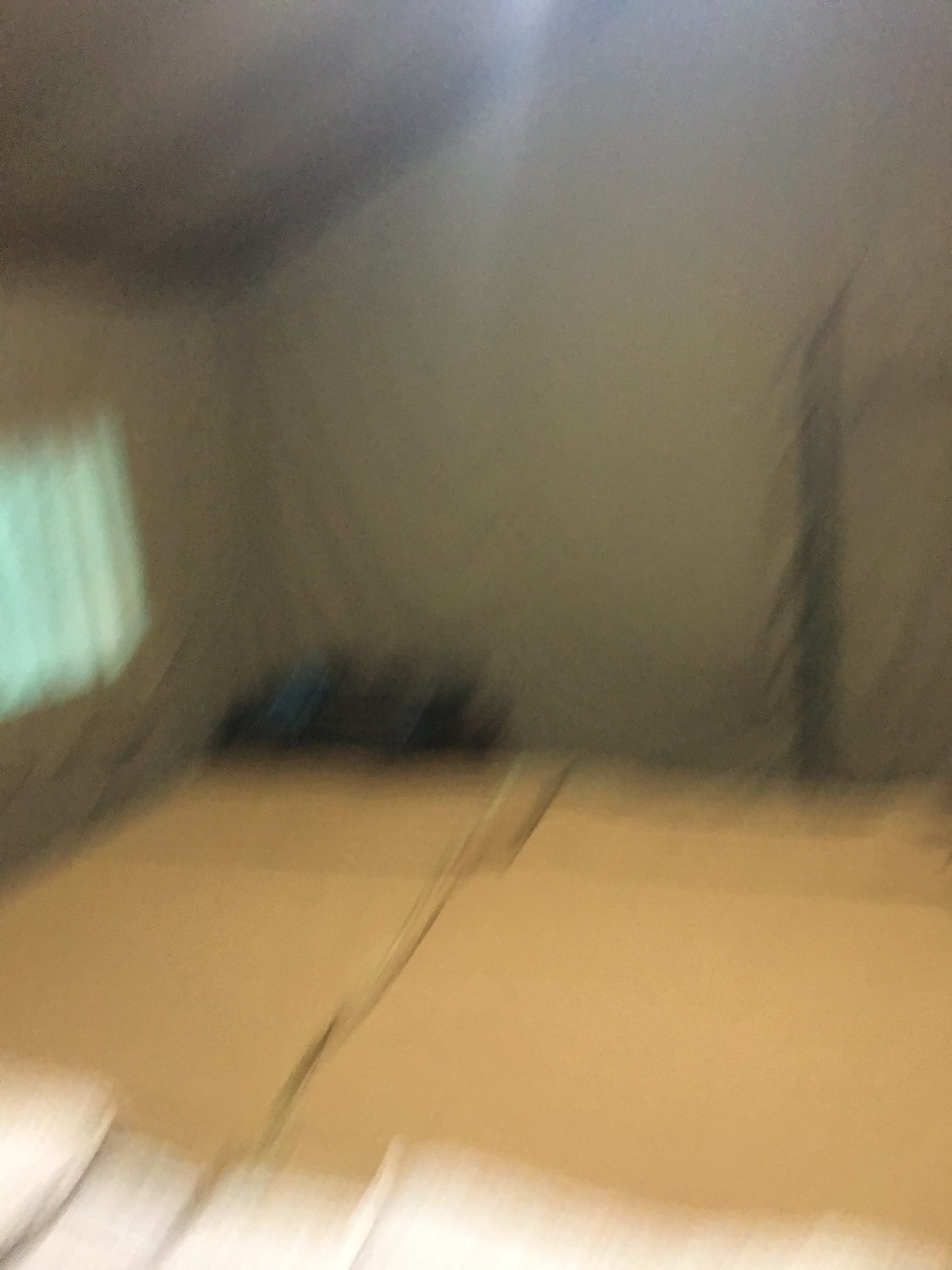This photograph captures the interior of a room undergoing renovation. The floor is covered with numerous light brown cardboard sheets or boxes, suggesting that protective measures are being taken during the construction process. Surrounding the room, the walls are draped with dark brown or possibly dark gray sheets, giving an impression of makeshift barriers or dust protection. On the left side of the image, a window can be discerned, with daylight filtering through the covering material, adding a soft, diffused light to the space. The room is characterized by its high ceiling, enhancing the sense of spaciousness. On the right side, a faint outline of a door is visible, hinting at an entry or exit point. Overall, the scene is indicative of ongoing renovation efforts, aimed at transforming the space.